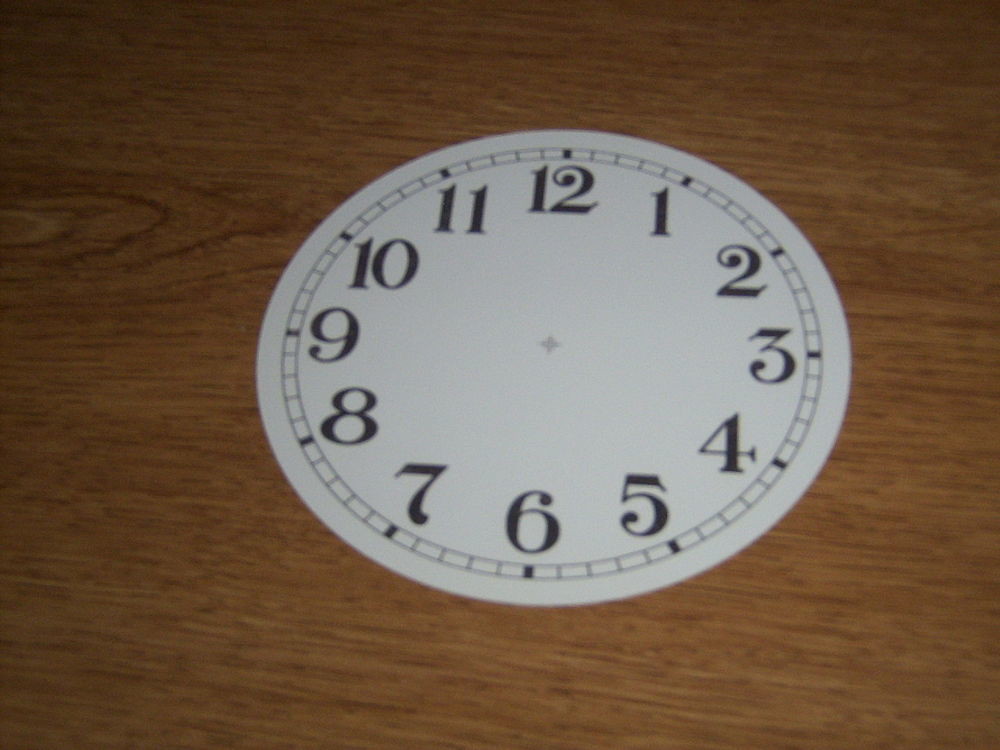The photograph features a wooden table, possibly made of formica, which serves as the backdrop. The table, which could be from a school or kitchen setting, is the subtle canvas for the main subject of the image: a white, round clock face. This clock face, adorned with an elegant font for the numbers, appears to be a component meant for a larger, possibly antique clock, such as a grandfather clock. The clock face is devoid of the clock hands and any other mechanisms, presenting only the numbered dial, perfectly round and seemingly poised to be integrated into a complete clock.